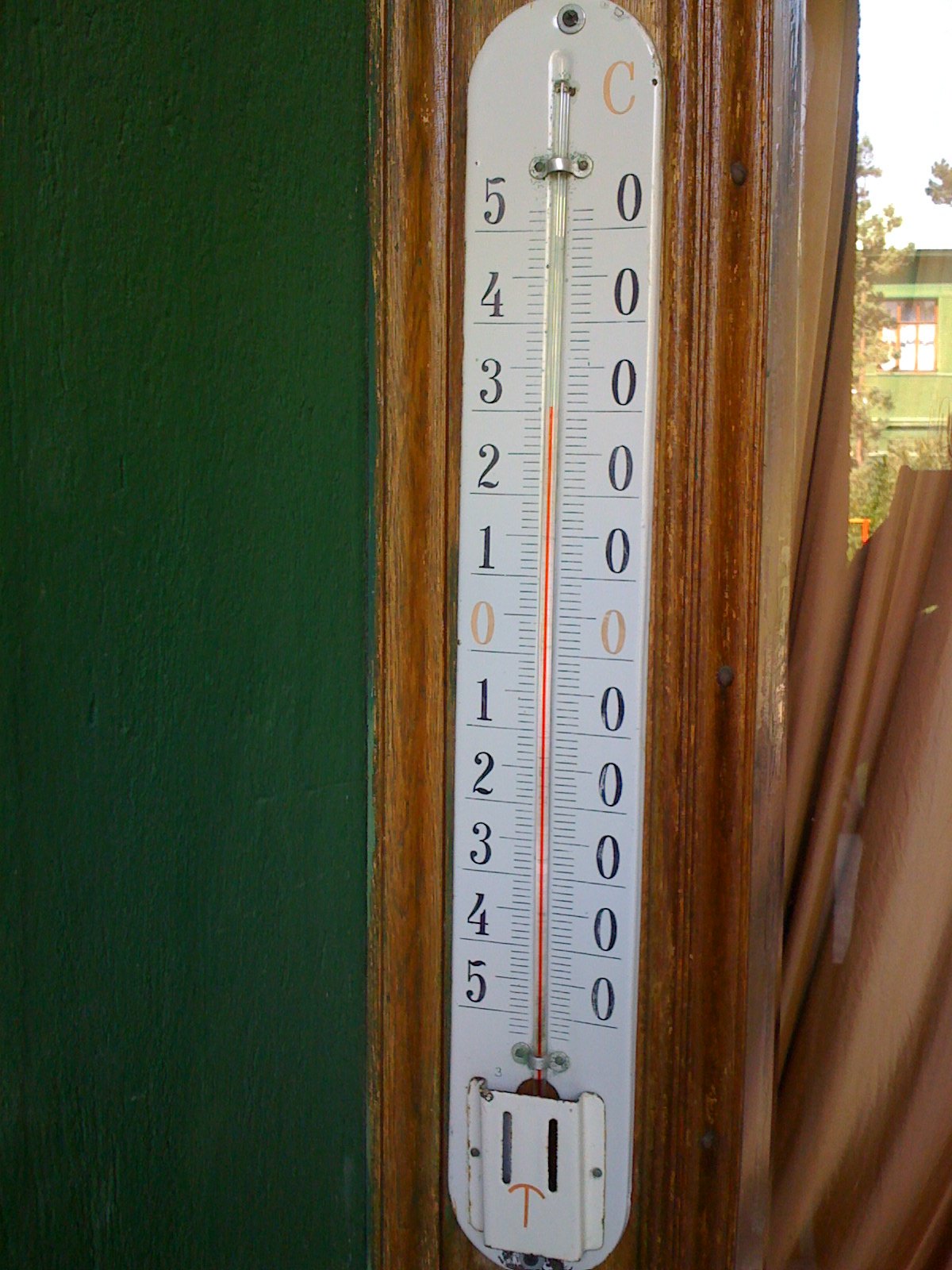Securely fastened to a brown wooden door frame, there's an alcohol thermometer displaying a detailed and somewhat unconventional design. This thermometer, painted white, features a back plate made of stamped metal. A notable detail is its unique numeric arrangement: on the left side, a column displays the tens place numbers, while on the opposite side, the zeros representing the ones column are shown. 

The temperature scale ranges from minus 50 to plus 50 degrees Celsius. Most of the numeric text is black, except at the zero mark, where faded text suggests the original red color, now appearing slightly orange. Positioned at the base of the thermometer is a protective cover that encases the sizable red fluid-filled bulb, with the fluid level currently indicating a temperature of around 31 degrees Celsius—a notably high reading.

Adjacent to this setup, the wooden door frame contrasts with a dark green painted wall. Beyond the doorway, the image captures a fleeting glimpse of the outdoors, featuring an overexposed view of a neighboring house with a visible window. The overall scene merges utility with a distinct, charming visual presentation.